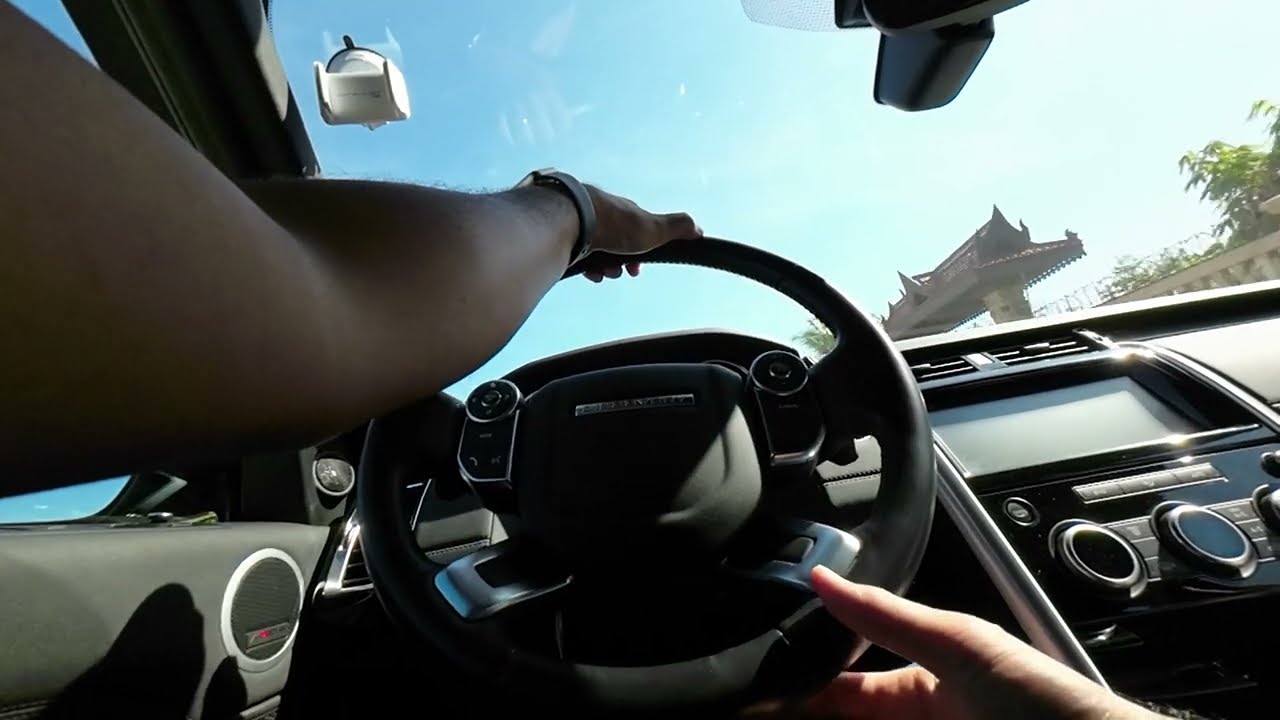The image provides a detailed point-of-view perspective from a driver inside a vehicle. The black steering wheel, adorned with silver markings and buttons on either side of its center, is held by the driver—likely a female, inferred by the appearance of her fingernails. Her left hand grips the top of the wheel, where she wears a watch on her wrist, and her right hand is positioned at around the 5 o'clock mark on the wheel. The angle of the photo suggests it was taken from the driver’s lap or stomach.

Inside the vehicle, the black interior is noticeable, with a visible center console featuring several knobs, buttons, a screen, and air vents. The dashboard extends out to meet the windshield, where the mount for the rearview mirror is partially visible, along with another white suction-cup holder attached to the windshield, currently empty.

Looking outside the vehicle, the scene includes a clear blue sky and some green trees. To the right, there is a large building with an East Asian temple-style roof, adding an intriguing architectural element to the view. There's also a white wall running along the side with some greenery. Further ahead, there's a bridge under construction that abruptly ends within the field of view.